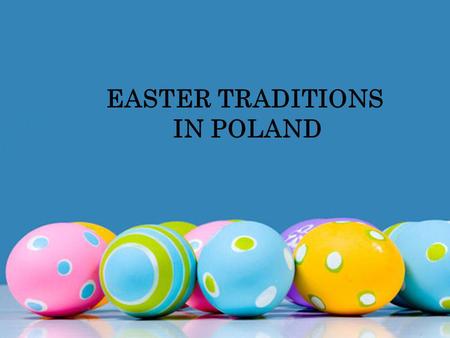The promotional poster for "Easter Traditions in Poland" features a dark blue background with the title prominently displayed at the top in black lettering. At the bottom of the image, a variety of intricately decorated Easter eggs are arranged on a reflective white surface, reminiscent of a shiny countertop. In the foreground, a vivid pink egg with white and blue spots stands out. Next to it, there is a blue egg adorned with white and green swirled stripes, and another blue egg with white and green dots. A yellow egg with similar white and green dots adds to the colorful display. Behind these, partially visible, is a purple egg with delicate white flower patterns and another pink egg with blue and white dots. In the very back, a green egg without visible markings and another yellow egg complete the festive array. The eggs, appearing in a few rows, are painted in various styles and colors, showcasing the rich tradition of Easter egg decoration in Poland.